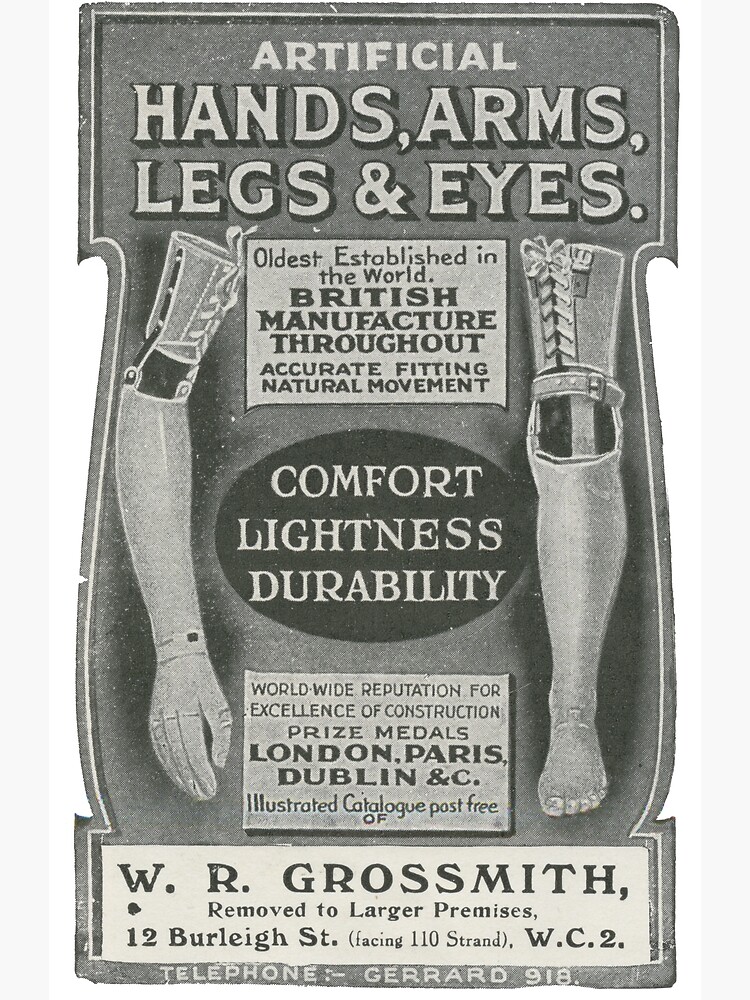This is a meticulously detailed black-and-white scan of an old advertisement poster. At the top center, it prominently reads in large white letters: "Artificial Hands, Arms, Legs, and Eyes." Below this header, the content narrows and features a detailed description extolling the company's virtues: "Oldest Established in the World British Manufacturer Throughout Accurate Fitting, Natural Movement, Comfort, Lightness, Durability." The ad emphasizes the company's "Worldwide Reputation for Excellence of Construction" and highlights "Prize Medals" won in London, Paris, and Dublin.

Flanking this text on both sides are intricate illustrations of a mechanical arm on the left and a mechanical leg on the right. Each appears segmented, showing various components such as the attaching straps, joints for the knee and elbow, and the movable hand and foot. Centered between these illustrations is a striking black oval with white lettering that reads: "Comfort, Lightness, Durability."

At the bottom of the poster and widening out slightly, more detailed information is provided in a white rectangular box. It states: "W.R. Grossmith" with a note indicating a move to larger premises at "12 Burleigh Street, facing 110 Strand, W.C.2." Additionally, the contact detail "Telephone: Gerard 918" is listed at the very bottom of the ad. This historical advertisement is both a testament to early prosthetic innovation and a visually intriguing piece of commercial art.